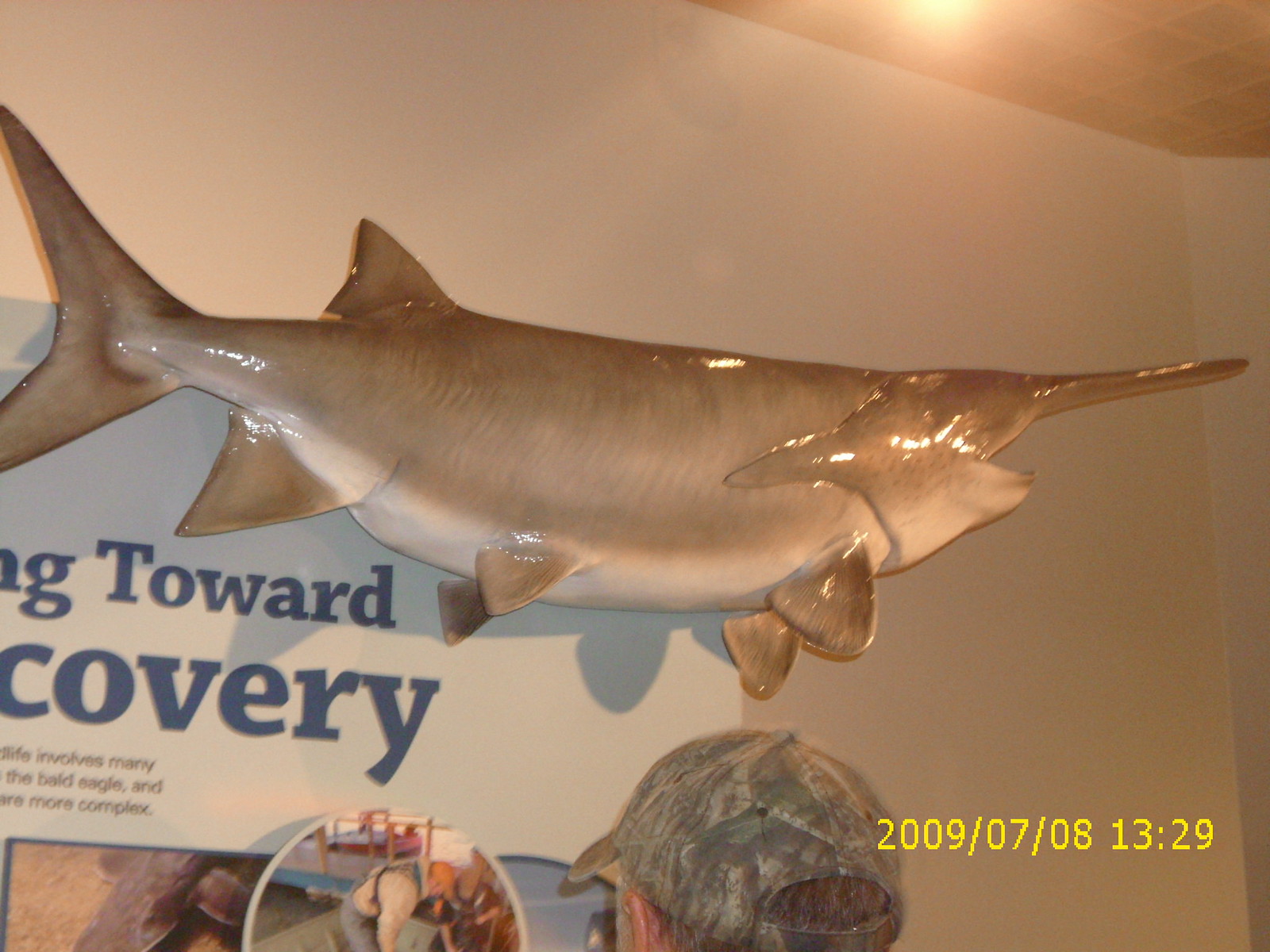This indoor color photograph, taken on July 8, 2009, at 1:29 PM and time-stamped in yellow numbers, features a large mounted fish, potentially a hammerhead shark due to its distinctive long bill. The fish, which appears either taxidermied or modeled, has a shiny beige and white coloration. It is mounted on a white wall above a sign with partially legible blue text that reads "Toward Recovery," indicating a display related to wildlife conservation. Beneath the fish and the sign, the top half of a man's head is visible; he is wearing a camouflage baseball cap and intently observing the exhibit. The background includes brownish ceiling tiles and a light fixture shining from the top right-hand corner.